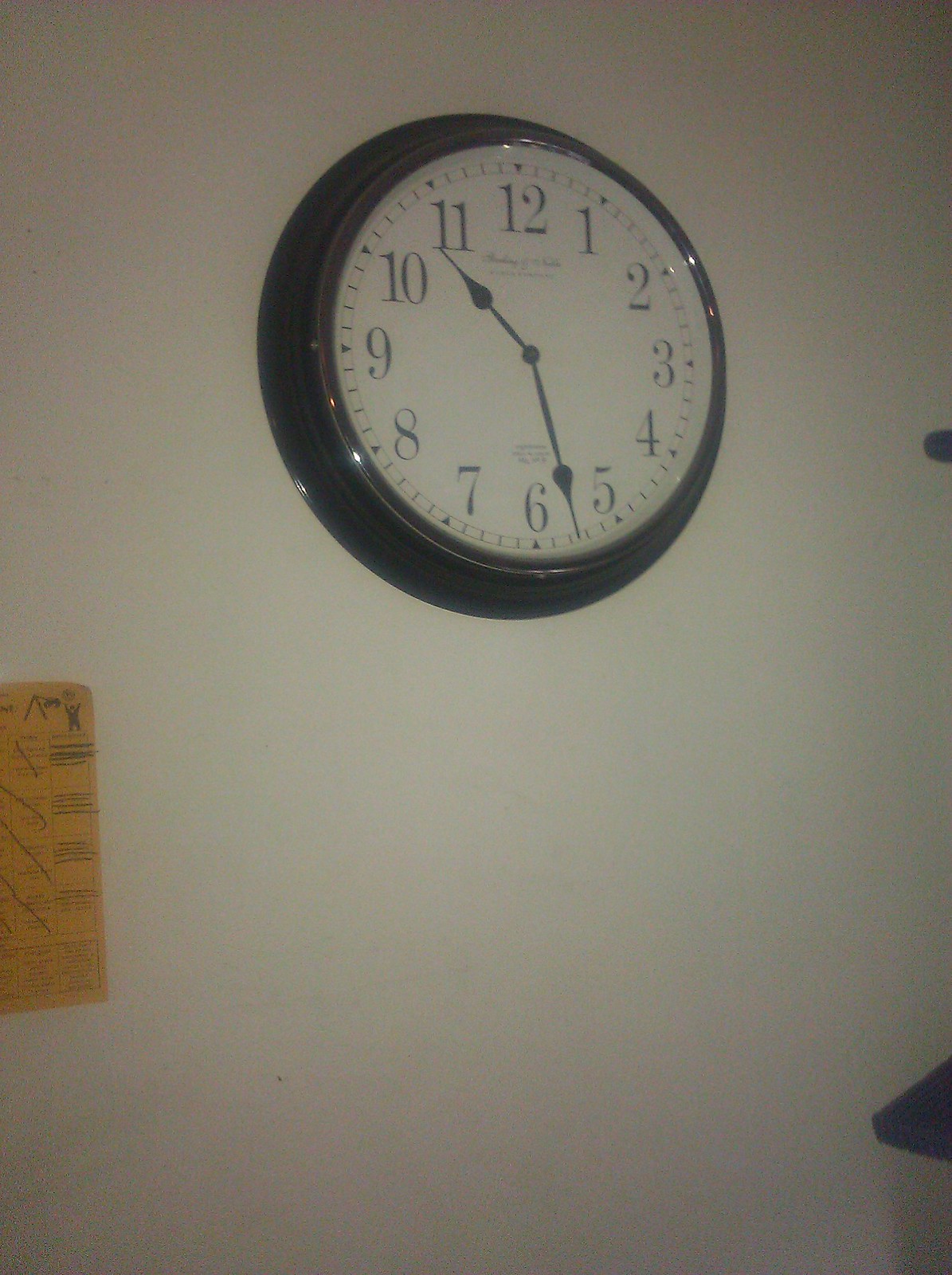This is a slightly blurry, low-lit color photograph of a round wall clock with a black or navy blue plastic frame that features an ornate, ribbed edge resembling crown molding, which flares out at the wall edge. The clock is mounted on a white wall. Its large, white face is clearly visible, displaying black numbers from 1 to 12, with every five-minute mark indicated by a black triangle. The minute and hour hands are black, ornate, and teardrop-shaped. The clock does not have a second hand and reads approximately 10:27 or 10:28. Light reflects off the glass covering the clock and the shiny frame, with noticeable reflections at the 12, 2, and 8 o'clock positions. Below the 12, there is some writing, possibly the clock's brand name, and additional text just above the 6. To the left of the clock, an orange piece of paper with black writing, possibly a calendar with crossed-off days, is tacked to the wall. On the lower right, a small section of a brown shelf edge is visible, and higher up, a blue triangular nubbin and a small blip poke out, adding subtle details to the scene.